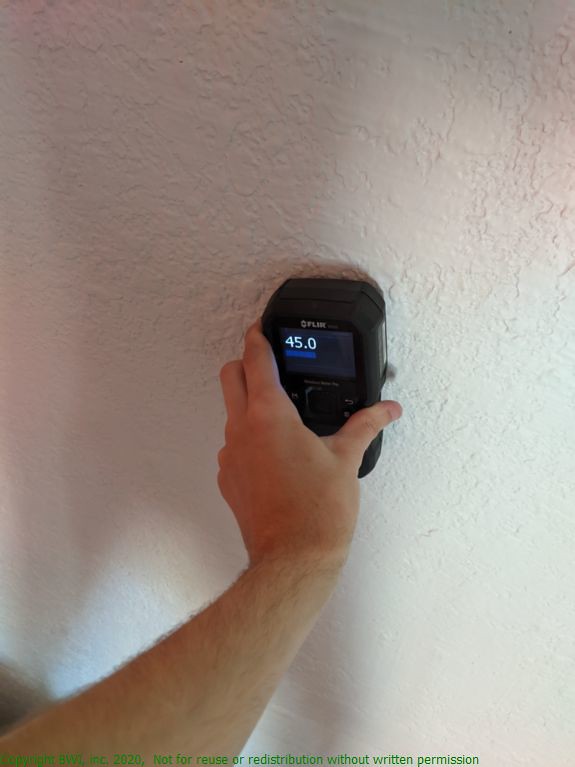In this photograph, a man is depicted attempting to locate a stud behind a textured, white-painted wall using a stud finder. The scene appears to be set in a hallway, though the image is cropped closely, focusing solely on the wall and the subject’s arm. The man’s left forearm extends into the frame from the left-hand corner, with his hand positioned towards the center. His hand is holding a black, rounded, rectangular stud finder, with the brand name "FLIK" (spelled F-L-I-K in white, capital letters) clearly visible at the top. The device features a digital display showing the measurement "45.0," accompanied by a blue horizontal bar underneath. Notably, the wall's textured surface suggests a stucco finish. At the bottom of the photograph, there's a printed disclaimer stating, "Not for reuse or distribution without written permission."